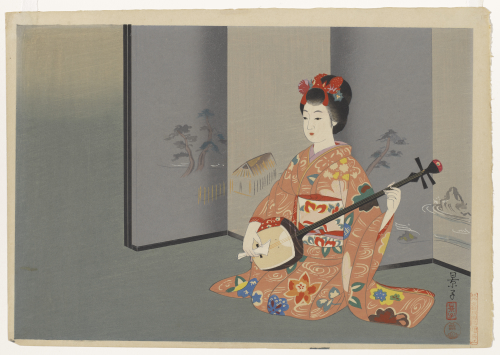This vintage Japanese woodblock style painting depicts a traditional woman playing a stringed instrument. She is gracefully seated on her knees, positioned in front of a four-panel folding screen used for privacy. The screen panels are decorated with intricate paintings of houses, trees, and white cresting waves, arranged in alternating shades of dark bluish-gray and light gray. The woman wears a striking orange kimono adorned with green and orange floral patterns. Her black hair is elegantly styled in a bun, embellished with flowers, a red bow, and other colorful decorations. She holds a unique guitar-like instrument with a rounded top and bottom, using a large paddle-like pick in her left hand, while the thin neck of the instrument, featuring a distinctive red ball at its top, stretches across her lap. The background of the artwork transitions from a subtle bluish-gray to a beige-brown gradient, adding depth to the scene. In the bottom right corner of the painting, there are vertical Japanese characters, with two black symbols above two red ones, alongside a watermark. The entire scene is set against a softly textured backdrop, bringing a timeless quality to this exquisite portrayal of Japanese culture and artistry.